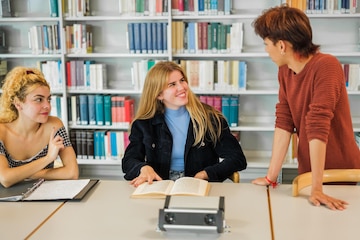In a cozy library or study area, three young individuals are engaged in an animated discussion. A boy, wearing a rust sweater with the sleeves pushed up, stands to the right, speaking to two girls who are seated. The boy appears younger than the two girls, adding a dynamic contrast to the scene. The girl with straight, long hair, dressed in a dark jacket over a light blue shirt, smiles broadly, her hand poised to turn a page in the open book before her. The second girl, with curly long hair, has an open binder with a notebook inside in front of her, and she too looks at the boy, smirking slightly. Behind them, a well-stocked bookcase laden with books enhances the studious atmosphere, making the scene reminiscent of a clip from a television program or movie.